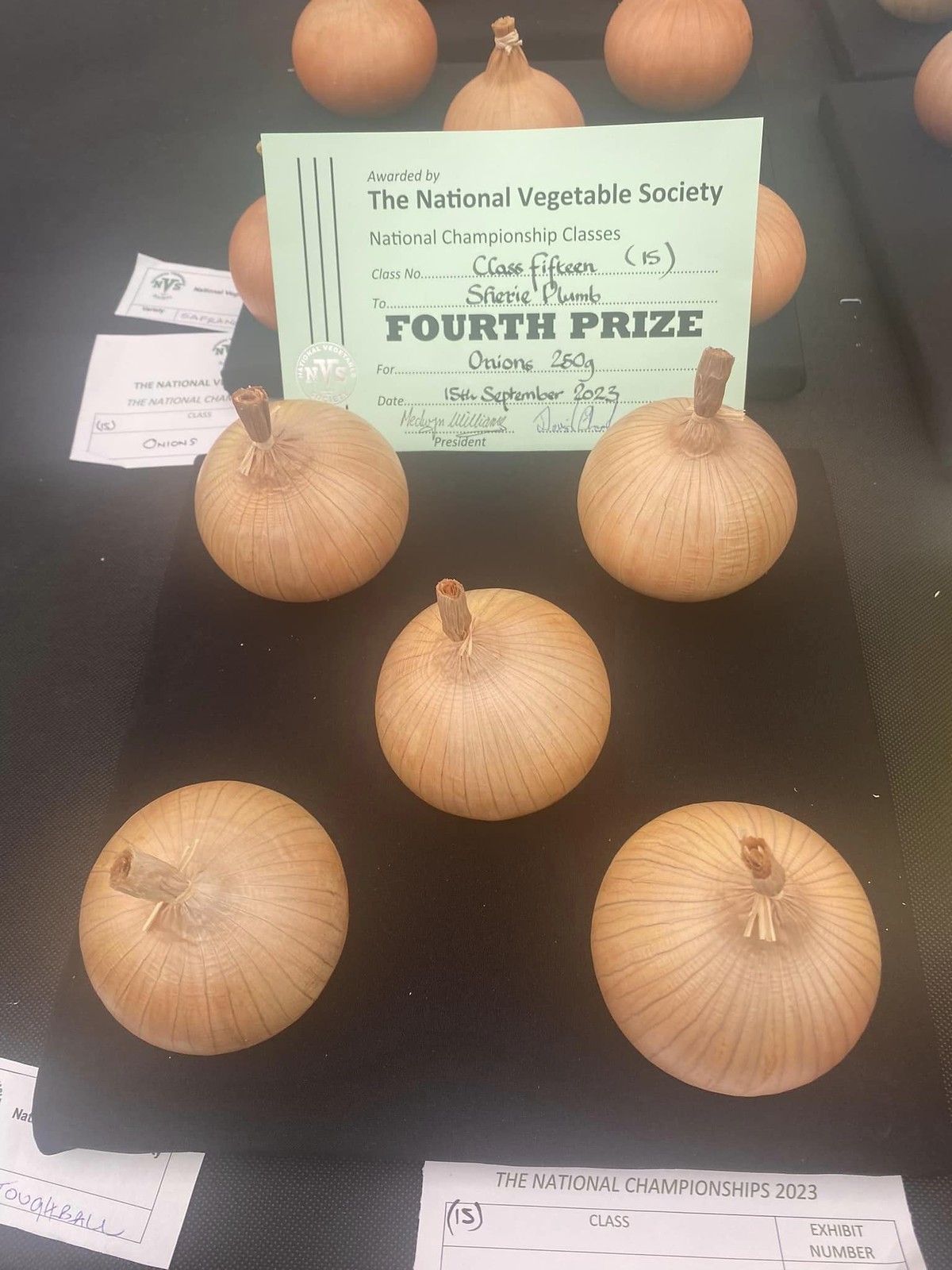In the image, there is a black-top table featuring a display of five uniformly shaped, light brown onions, arranged in a pattern similar to the five-face of a die. On the table next to these onions is a prominent white sign containing detailed information written in black text. The sign, which has three parallel lines running from top to bottom on the left side, reads: "Awarded by the National Vegetable Society. National Championship Classes. Class number 15." The number "15" is additionally shown in parentheses. Below, the text states: "To Sheree Plumb. Fourth prize for onions. 250 grams. Date: 15 September 2023." This is followed by a name and a signature, accompanied by the title "president." In addition to this main set of onions and the sign, there appears to be another identical set of five onions arranged behind the sign, potentially part of a separate entry on the same table. The card also features a detail in light green color, adding to the official look of the proclamation. Congratulations to Sheree Plumb for her award-winning onions.